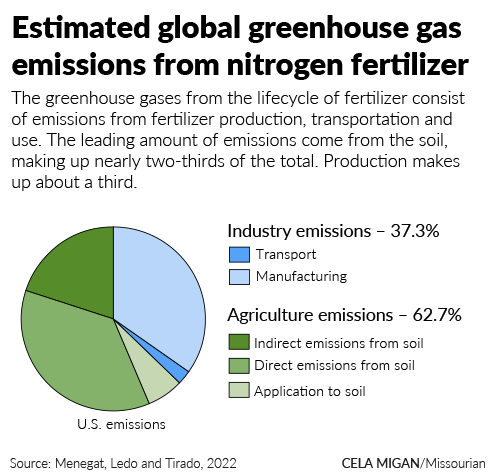This infographic titled "Estimated Global Greenhouse Gas Emissions from Nitrogen Fertilizer" illustrates the breakdown of emissions from various sources associated with nitrogen fertilizer. Dominating the image, the pie chart on the left is layered in colors from light blue to dark green, each representing different sources of emissions within the U.S.

The largest segment of the pie chart, covering almost two-thirds (62.7%), is related to agricultural emissions, broken down further into direct emissions from soil, indirect emissions from soil, and application to soil. Direct soil emissions form the bulkiest part, nearly 40%, with indirect emissions from soil around 20%, and application emissions covering the remainder.

On the right, industry emissions are detailed, constituting 37.3% of the total. These industry emissions are split into manufacturing and transport, with manufacturing being the majority share, indicated though specific percentages aren’t provided.

The infographic also references its sources: "Menegat, Lado, and Tirado, 2022" and mentions "Sila, McGann, Missourian," possibly linked to its publication.

Overall, the chart visually communicates the predominant contribution of soil-related agricultural activities to greenhouse gas emissions from nitrogen fertilizer, with production and transportation sectors also making significant contributions.